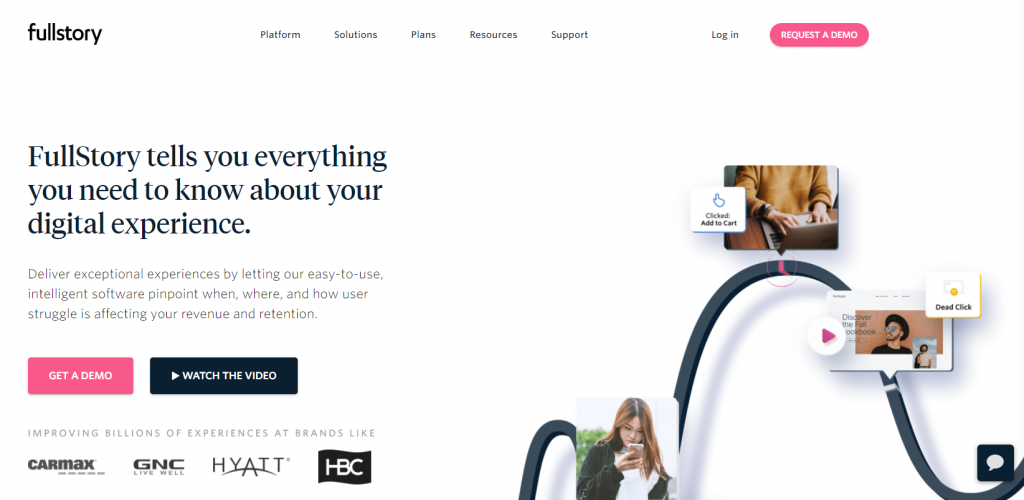The top section of the website features a predominantly white background. On the left-hand side, the heading "Full Story" is displayed in bold, followed by a navigation menu in black text listing the options: Platform, Solutions, Plans, Resources, and Support. To the far right, the options "Login" and a pinkish oval button with "REQUEST A DEMO" in white, capital letters are visible.

Below this, the bold heading "Full Story tells you everything you need to know about your digital experience" is prominently displayed. The accompanying subtext reads, "Deliver exceptional experiences by letting our easy-to-use, intelligent software pinpoint when, where, and how your users' struggles are affecting your revenue and retention."

Two call-to-action buttons are positioned beneath the text: a pink one with "GET A DEMO" in white, capital letters, and a black one labeled "WATCH THE VIDEO." Adjacent to them, a white rectangle on the left side provides a visual contrast.

Underneath, in smaller gray text, the statement "Improving billions of experiences at brands like" introduces a list of brands: CarMax, GNC Live Well, Hyatt Hotels, and HBC.

On the right side, three images are arranged vertically: the first depicts a girl looking down at her phone, the second shows two hands typing on a black and silver laptop, and the third features a man looking up at the sky while wearing sunglasses.